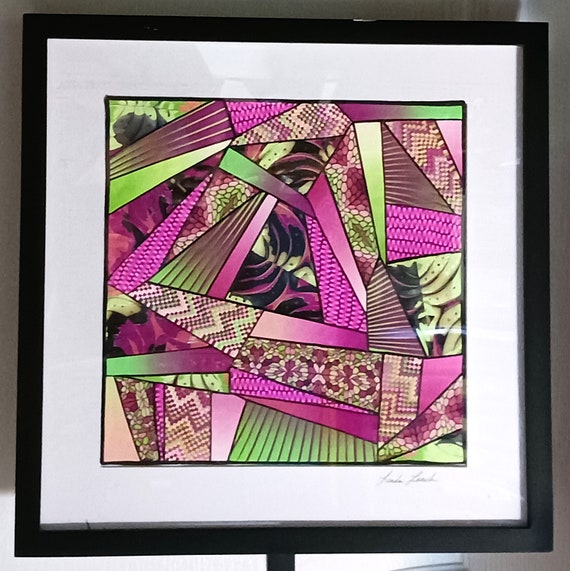This image showcases a framed print of an abstract painting. The black frame encases a white background that surrounds the main artwork, with a cursive signature of the artist in the bottom right corner. The centerpiece of the artwork is composed of a patchwork of various geometric shapes, predominantly triangles, rhombuses, and disproportionate rectangles. These shapes are filled with intricate patterns, such as green vertical stripes, pink frilly stripes reminiscent of fish scales, and floral stained glass motifs. The vibrant color palette includes shades of lime green, hot pink, dark purple, red, brown, and black, creating a harmonious yet dynamic visual experience. The entire framed piece is set against a grey backdrop.